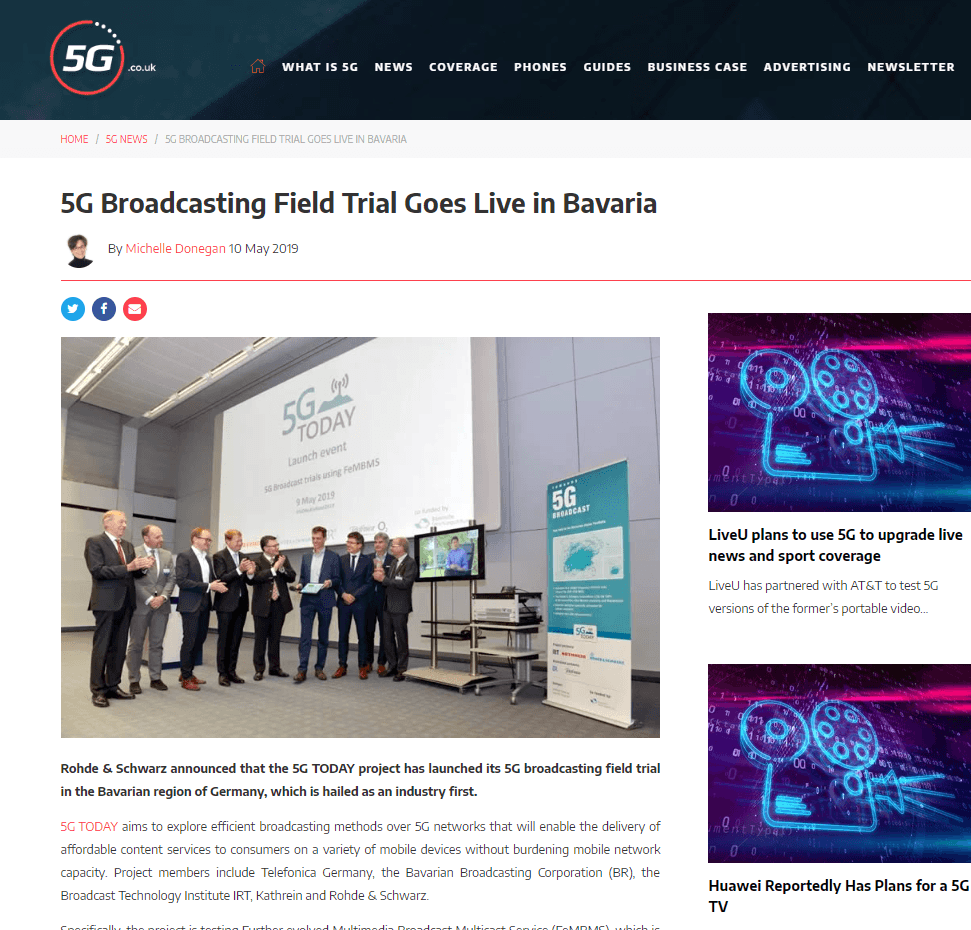This is a webpage from 5G.co.uk featuring a thick black banner across the top. On the far left, it displays the 5G logo in bold white text encircled by a red ring that transitions into several white dots to complete the circle. To the right of the logo, bold white capital letters list various sections: "What is 5G?", "News", "Coverage", "Phones", "Guides", "Business Case", "Advertising", and "Newsletter". 

Beneath this, a thin, pale gray banner spans the width of the page, presenting navigation options from left to right: "Home", "5G News", and "5G Broadcasting Field Trial Goes Live in Bavaria", with the latter option highlighted as the current selection.

In the main content area against a white background, the article title "5G Broadcasting Field Trial Goes Live in Bavaria" appears in bold black text. Underneath, an author's avatar is displayed alongside the byline "By Michelle Donegan, 10 May 2019", with her name highlighted in red. 

There are three icons for connecting with the company on social media: Twitter (X), Facebook, and email. Below this, a photograph shows several men standing in a line, all wearing suits and smiling. A younger man in the center, dressed in a more trendy fashion, holds a clipboard or a document, drawing the attention of the others. The setting appears to be a conference room with gray carpet, large gray tiled walls, and a ceiling outfitted with long tracks of fluorescent lighting. A screen in the background displays information about the "5G Today launch event".

The photograph's caption in black text reads: "Rode and Schwartz announced that the 5G Today project has launched its 5G broadcasting field trial in the Bavarian region of Germany, which is hailed as an industry first." The article then continues to discuss these developments in further detail.